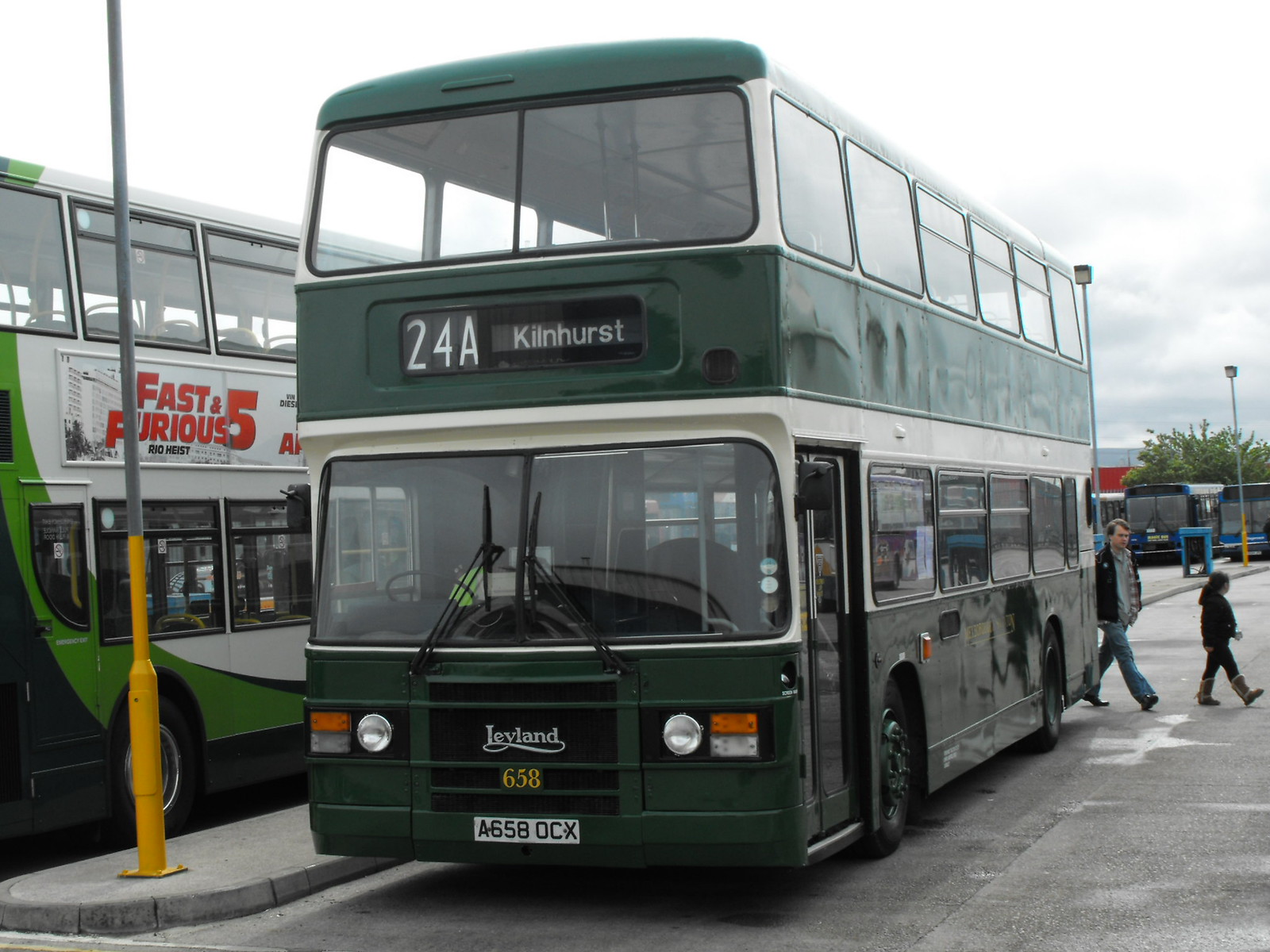In this bustling bus depot on a gray, overcast day, a classic dark forest green double-decker bus, identified as a Leyland 658, sits prominently. Its route is marked as 24A to Kilmhurst. This old-fashioned bus, seemingly from the 1970s, stands out with its lack of a front door and its vintage charm. Behind it, a man and a child cross the street, hinting at the daily activity in the area. To the left, a more modern double-decker bus, adorned with a vibrant "Fast and Furious 5: Rio Heist" design in white, lime green, and black swirls, contrasts sharply against the older model. This bus, likely from the 2000s, showcases the evolution of buses over the decades. In the background, several single-level buses are parked, emphasizing the depot's function as a central hub for various public transport vehicles. The scene is further detailed with the green bus's license plate, reading A658-OCX, adding an additional layer of authenticity to this snapshot of urban transit life.